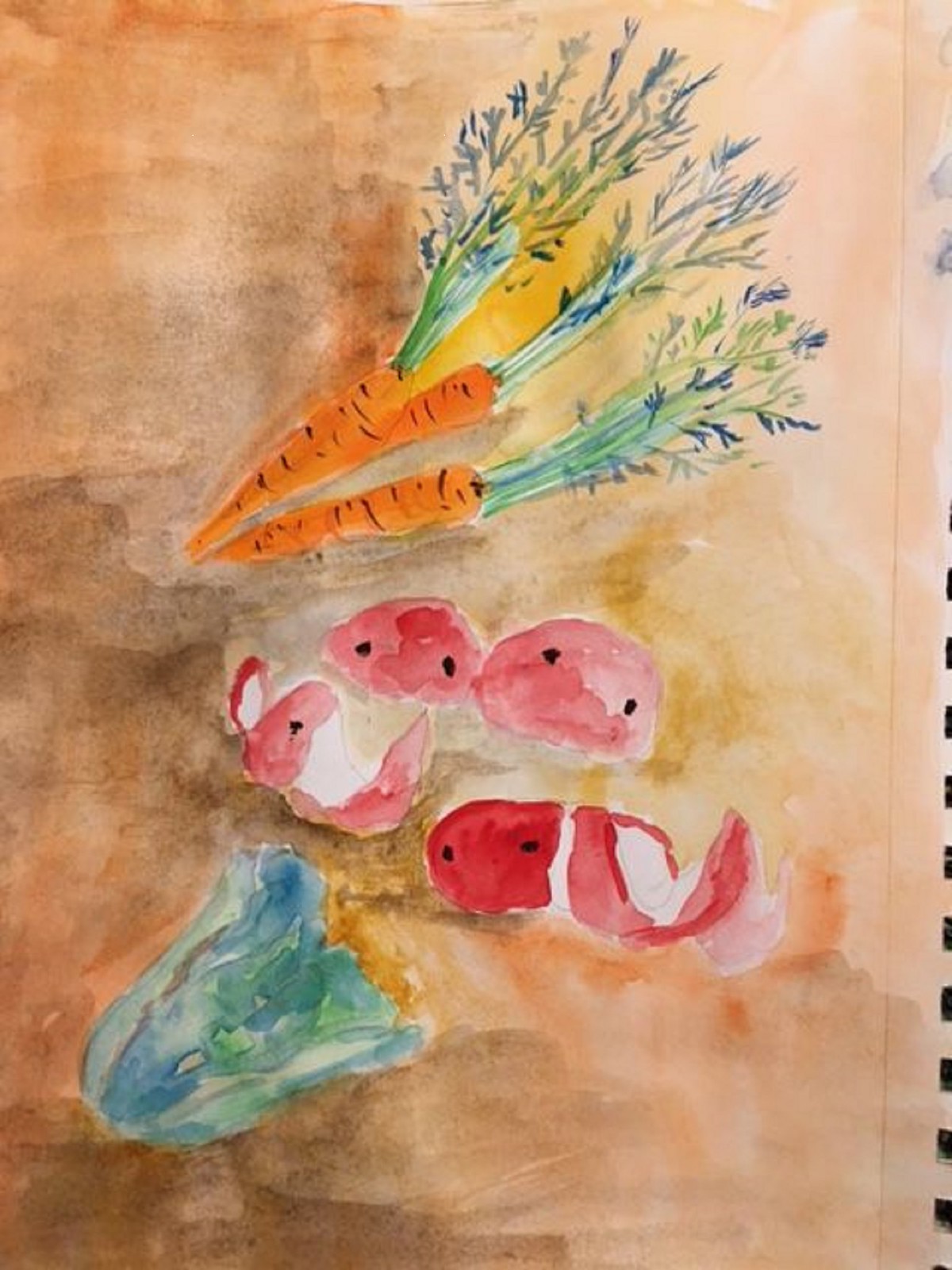The painting, created using watercolors, has a background predominantly composed of mixed shades of light and dark brown, with hints of red and yellow undertones. The image is viewed from a downward angle, resembling the perspective of looking at a page in a spiral notebook, indicated by visible holes along the bottom right corner. At the bottom of the painting, a green head of lettuce is depicted. Above the lettuce, there are peculiar red objects, featuring two black dots each, reminiscent of certain types of fruit or mushrooms, though their exact nature is ambiguous. These red elements are joined by additional pink, white, and blue circular shapes with black dot details, possibly representing mushrooms or flowers. Most notably, three carrots with distinct black lines and green stems crowned with leafy toppings dominate the upper section of the painting. Small blue stick-like protrusions can be seen emerging from the green stems, adding a unique element to the depiction. The combination of these detailed features creates a vivid and intricate watercolor composition.